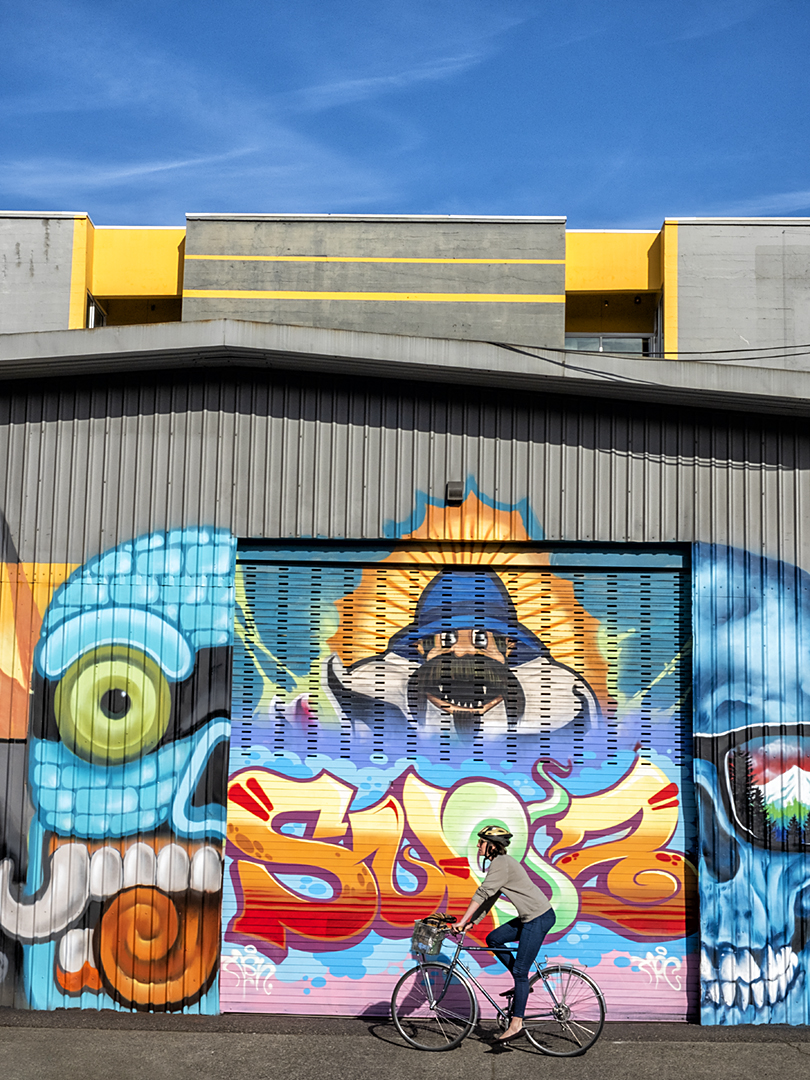The image captures a vibrant street scene with a clear blue sky above. In the foreground, a woman on a bicycle, wearing jeans, a sweater, shoes, and a helmet, rides past a large, graffiti-covered gray warehouse building with paneling on its walls. The graffiti mural features several colorful characters. On the right side, there's a blue skeleton with thick black glasses that depict a mountain scene with clouds, sticking its tongue out with one curved molar and large green eyeballs.

In the middle of the mural, there’s a character resembling a fisherman, wearing a wide-brimmed hat and sporting a prominent handlebar mustache. His eyes are bugging out, and his mouth is open wide, resembling a hawk's. Behind him, sun-like rays emanate upward, adding a dynamic background element.

To the left side of the mural, another cartoonish blue skull grins, showing distinct teeth, with exaggerated features and only its right eye visible. The graffiti is detailed, with bright yellow, orange, and red gradients, although the letters are mostly indistinguishable. Above the mural and the warehouse, the roof's eaves are visible, and in the background, additional buildings with yellow construction stripe patterns can be seen. The sky above is dotted with wispy, faded white clouds.